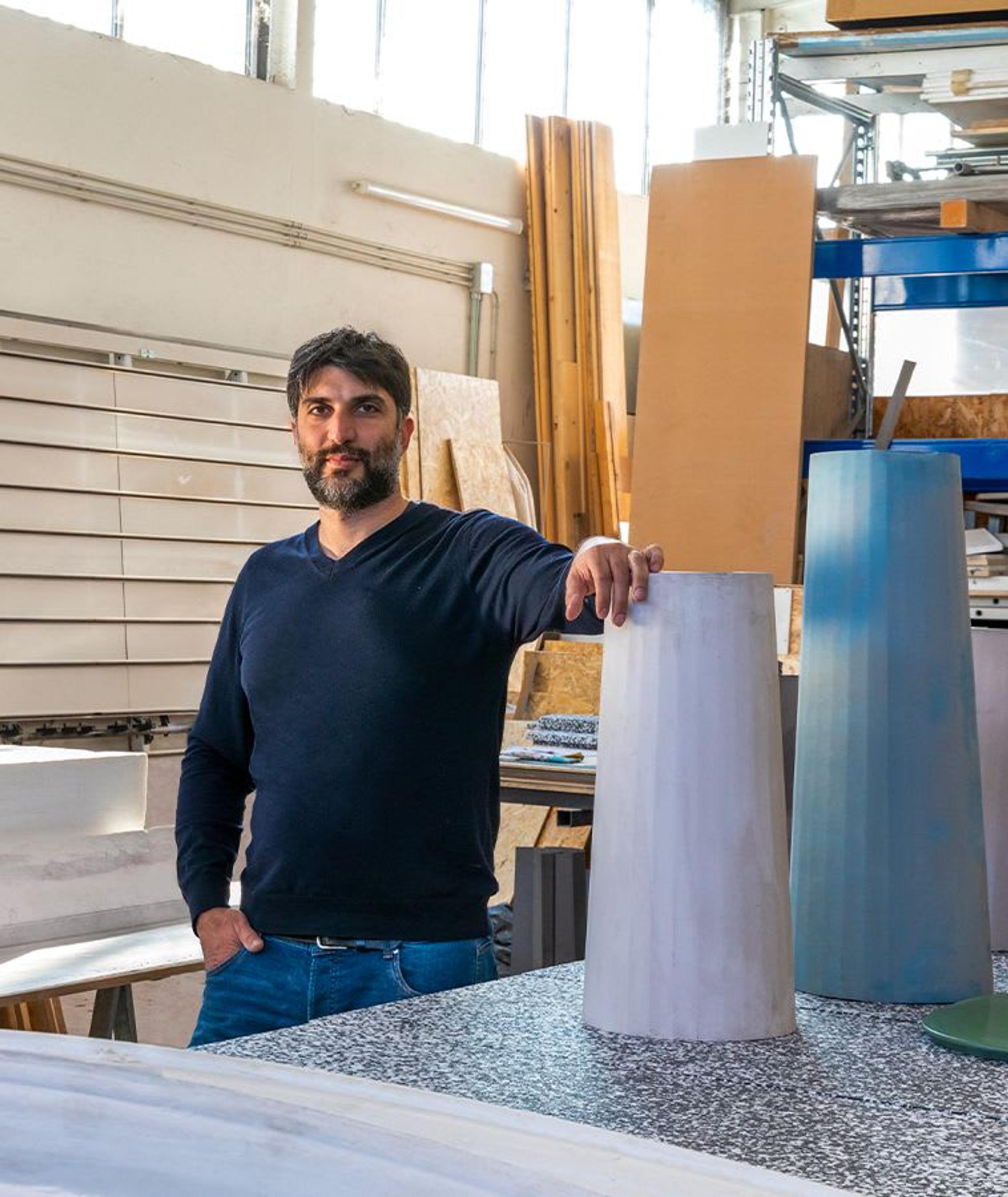In a vertically aligned rectangular picture, a man stands slightly to the left of center in a workshop-like room, dressed in a navy blue v-neck sweater over blue jeans. He has a composed expression, with dark brown hair that is shorter on the sides and combed neatly over his forehead. His facial hair includes a brown mustache, brown eyebrows, and a dark brown beard with hints of gray. His right hand rests in his front jean pocket, while his left hand is placed on top of a white cylindrical object resembling a narrow lampshade. Beside it, there is a taller light blue cylindrical object, both situated on a speckled gray and white countertop in the lower right corner of the image. 

In the background, a tan-colored garage door with horizontal slats is visible, topped by a tan wall. Above this is a large window composed of vertical rectangular panels, through which sunlight streams. The upper right corner reveals what appears to be a lumber yard, with long wooden planks stacked against the wall. There are also additional objects and a blue set of metal shelves along the back wall. The man's skin tone is relatively tan, and the overall scene is bathed in natural light coming from the window.